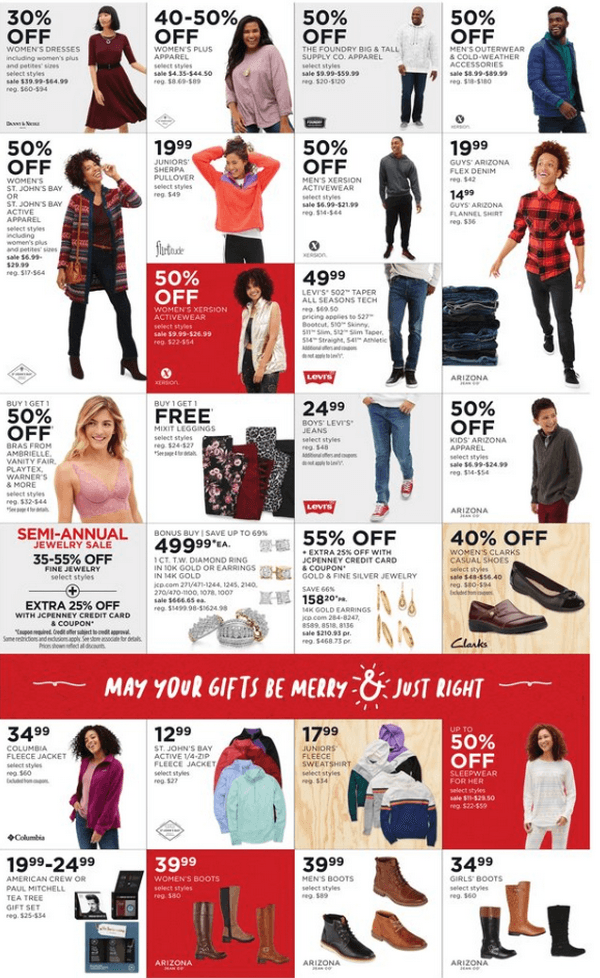**Caption:**

This is a detailed screenshot of a newspaper advertisement featuring a variety of discount offers for clothing and accessories. The top section displays a grid layout consisting of seven rows, each with four boxes. Key highlights include:

- A woman in a dress with a label offering 30% off.
- Next to her, a woman in a pink top is shown with a discount of 40-50%.
- A man wearing a white shirt is advertised at 50% off.
- A man in a blue jacket also available at 50% off.

A larger, rectangular box prominently features a woman in a plaid jacket. Adjacent to her, a woman in a red shirt is displayed. Below her, another box showcases a woman in a white vest.

The advertisement also includes multiple promotions for men's clothing, such as jeans, tops, and active wear, in addition to men's shoes. At the bottom, there are three ads focused on footwear, including separate offers for men’s and women’s boots, as well as girls' boots.

Other featured items include gift sets, fleece jackets, junior fleece sweatshirts, jewelry, and diamonds. A festive banner with the message "May Your Gifts Be Merry and Just Right" is also visible, along with an ad for women's sleepwear, showcasing a woman in a white outfit.